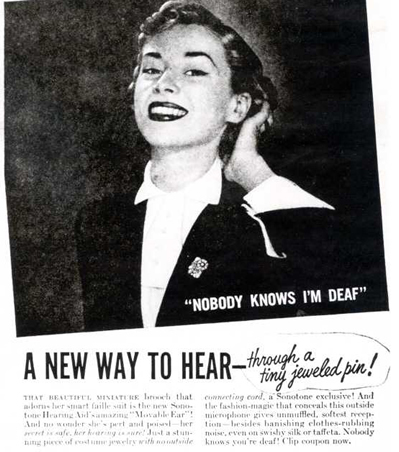In a striking black-and-white image evocative of the 1950s, a woman with a short, vintage hairstyle and dark makeup holds her left hand to her ear, as if showcasing a hearing device. She is adorned in a dark jacket featuring an emblem and a white shirt, complemented by her pronounced dark eyebrows and lipstick. Her expression is poised against a backdrop that reflects shades of black and gray. In the lower corner of the image, white text announces, "Nobody Knows I'm Deaf," followed by another message in black text that reads, "A new way to hear - through a tiny jeweled pin." The elegant cursive underlines the sophistication of the phrase, and additional explanatory text is subtly included below, blending with the background. This composition, possibly reminiscent of an album cover or an advertisement, seamlessly combines visual elements to emphasize the revolutionary hearing aid discreetly worn by the woman.